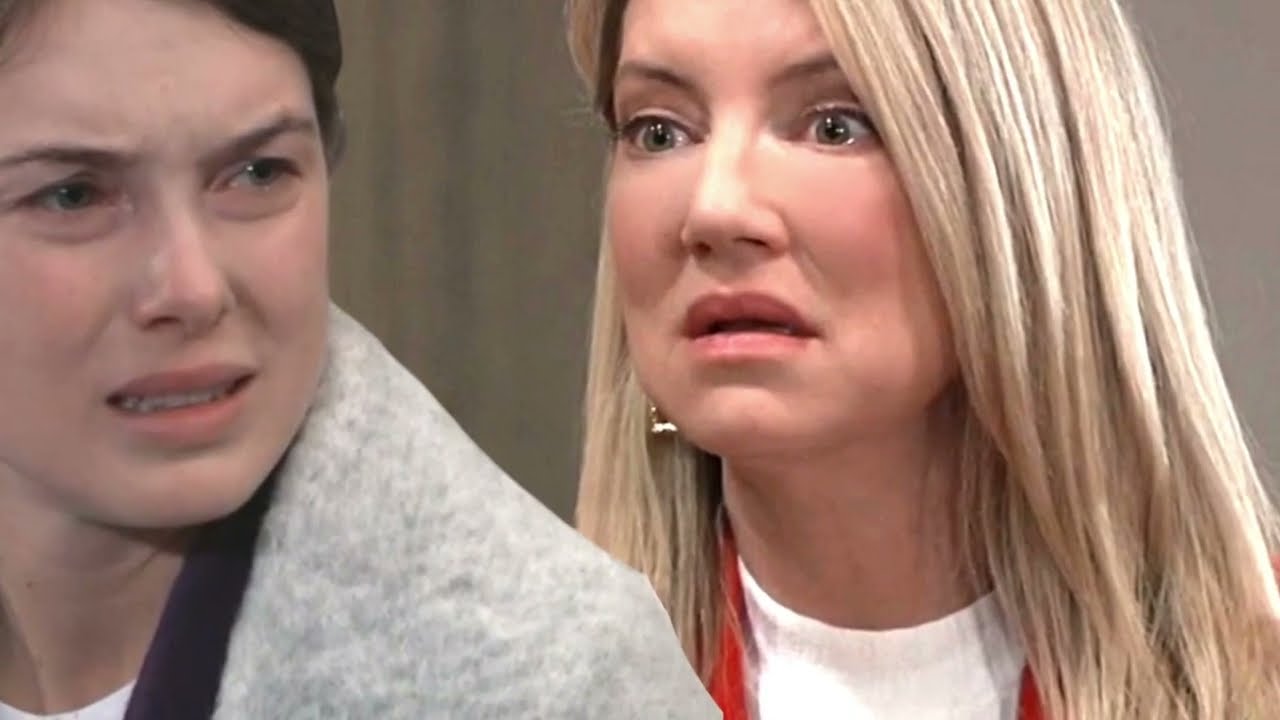This image features two women set against a brownish-gray wall, with one appearing to be superimposed over the other. The woman in the foreground has black hair tied back, blue eyes, and an expression of confusion or distress, with her mouth open and her eyebrows furrowed. She is wearing a gray hoodie or coat with a black trim around the neck. The woman behind her has long blonde hair framing her face, chubby cheeks, green eyes, and a downturned mouth that gives her an annoyed look. She is wearing earrings, a white t-shirt, and a red or orange jacket. This still frame, potentially from a movie or reality television show, lacks additional context but highlights the contrasting emotions between the two women.